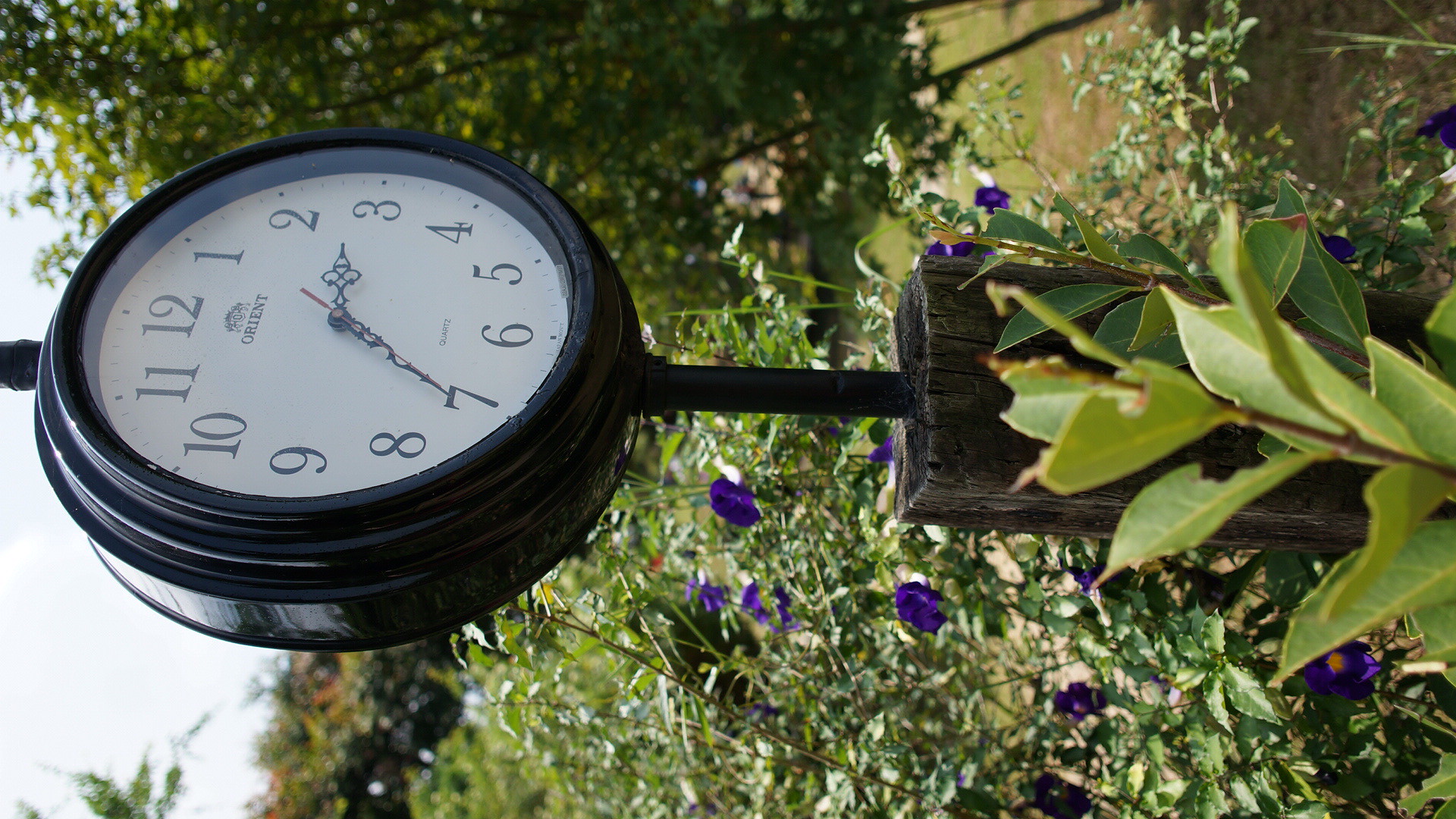This horizontal color photograph captures an artistic garden scene, although it has been rotated 90 degrees counterclockwise, positioning the top of the image to the left. At its heart stands a large, black metal clock with intricate detailing, mounted on a sturdy stand resting on a wooden surface. Surrounding the clock is a lush garden filled with an array of green leaves and vibrant purple flowers, adding a natural charm to the scene. In the background, a well-manicured lawn extends towards softly focused trees, creating a serene and picturesque setting.

The clock reflects sunlight, accentuating its polished metal surface. Dominating the clock face is a crisp white background with bold black numerals from 1 to 12 encircling the edge. Below the number 12, the brand name “Orient” is elegantly inscribed. The clock features ornate hour and minute hands, with a striking red second hand poised at the center. The time displayed is 2:35.